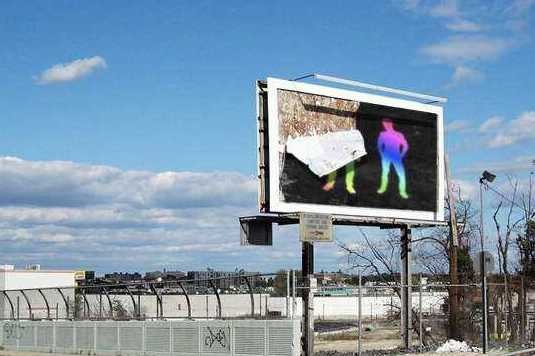In this outdoor photograph taken on a sunny day, we see a large, partially damaged billboard situated against a backdrop of a clear blue sky with some white, fluffy clouds scattered near the horizon. The image captures a city skyline in the distance, and the lower part of the frame includes a gray cement half-wall adorned with simple black graffiti. This wall is topped by a curved chain-link fence and features chain-link gates to the right. The billboard itself is framed in white and displays a black background with two vibrant, rainbow-colored silhouettes of dancing figures. The right figure remains intact, displaying a gradient of colors from pink at the top to blue and green toward the feet. However, the left figure is compromised, with the upper portion of the billboard art peeling and revealing a brown underside, leaving only the yellow-green legs visible. The area around the billboard includes additional gray walls and a series of tall light poles.